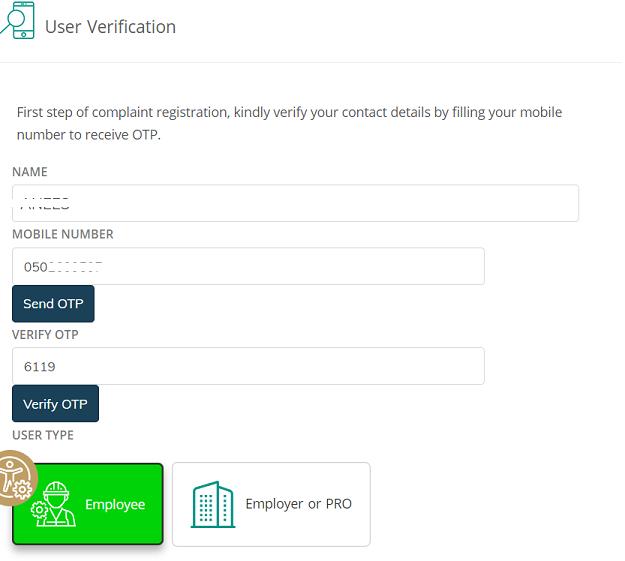The image is a screenshot of a user verification page, presumably from a security-focused interface. At the top, bold text reads "User Verification," accompanied by an image of a mobile phone with a magnifying glass overlay, symbolizing scrutiny or verification of sensitive information like secrets or passwords. 

Below, a message states, "First step of complaint registration: Kindly verify your contact details by filling in your mobile number to receive an OTP." 

The form on the page includes several text fields. The first field is labeled "Name," with an input box underneath it. For privacy, the actual name entered has been censored. The next field is for entering a mobile number, where the visible part reads "050," with the remaining digits obscured for privacy. Below this field, a button labeled "Send OTP" is visible.

The section that follows is for OTP (One-Time Password) verification. It includes a text box with the numerical code "6119" already entered. Below this, a button labeled "Verify OTP" is present.

At the bottom of the page, there are two distinct buttons. The first button reads "Employee" in white font set against a green background, featuring an icon of a person wearing a hard hat with a gear on their shoulder, suggestive of a worker or technician. Next to it, the second button reads "Employer or PRO" and is accompanied by an icon depicting an office building.

This detailed layout indicates a step-by-step process for verifying contact information, possibly as part of complaint registration or security validation.